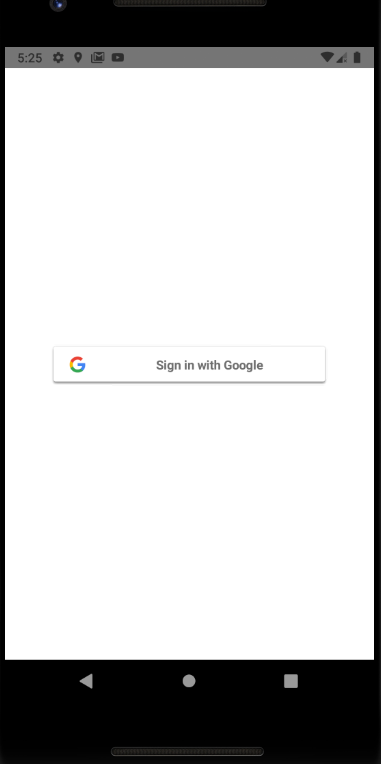The image displays an iPhone screen with a minimalistic interface. The iPhone is fully charged and shows a strong connection, as indicated by the icons in the light gray status bar at the top of the screen, alongside the time which reads 5:25. 

Below the status bar is a wider black strip that spans the top of the device. The main area of the screen features a clean, white background with no additional text or imagery, creating a stark and simple layout. Central to the screen is a prominent sign-in prompt that reads "Sign in with Google." This prompt is accompanied by the Google "G," which is beautifully rendered in Google's signature colors: red, yellow, blue, and green. The box containing the sign-in prompt nearly stretches across the entire width of the screen but leaves slight margins on either side.

At the bottom of the phone, a thick black strip runs from edge to edge, displaying navigation controls. The home button is situated centrally within this strip. To the left, there's a left-pointing arrow, and to the right, there's a gray square, likely for additional functionalities. The overall color scheme of the image is predominantly black and white, with the only splash of color coming from the Google "G" in the middle of the screen.